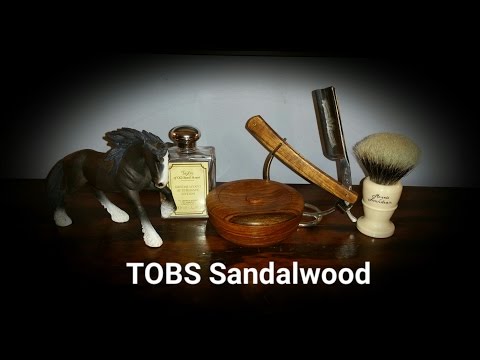The advertisement showcases an elegant array of men's grooming essentials centered on a polished wooden table, all set against a dramatic black background with a hint of a white circle at the center, creating a striking visual focus. Prominently featured on the left is a sophisticated glass bottle, likely containing cologne or aftershave, with "T.O.B.S. Sandalwood" inscribed at the bottom, endorsing the premium quality of the product. Adjacent to the bottle, a finely detailed horse figurine adds a classic masculine touch. To the right, a luxurious wooden bowl suggests a traditional shaving cream container, accompanied by a vintage-style shaving brush with a similarly polished wooden handle. Completing the scene on the far right, a straight razor with a wooden grip rests, hinting at an old-fashioned shaving ritual. Beneath the razor, an indistinguishable metallic tool peeks out, adding an element of intrigue. The meticulously arranged items, accentuated by subtle hues of brown, produce a nostalgic yet refined atmosphere, perfect for an advertisement targeting traditional grooming aficionados.